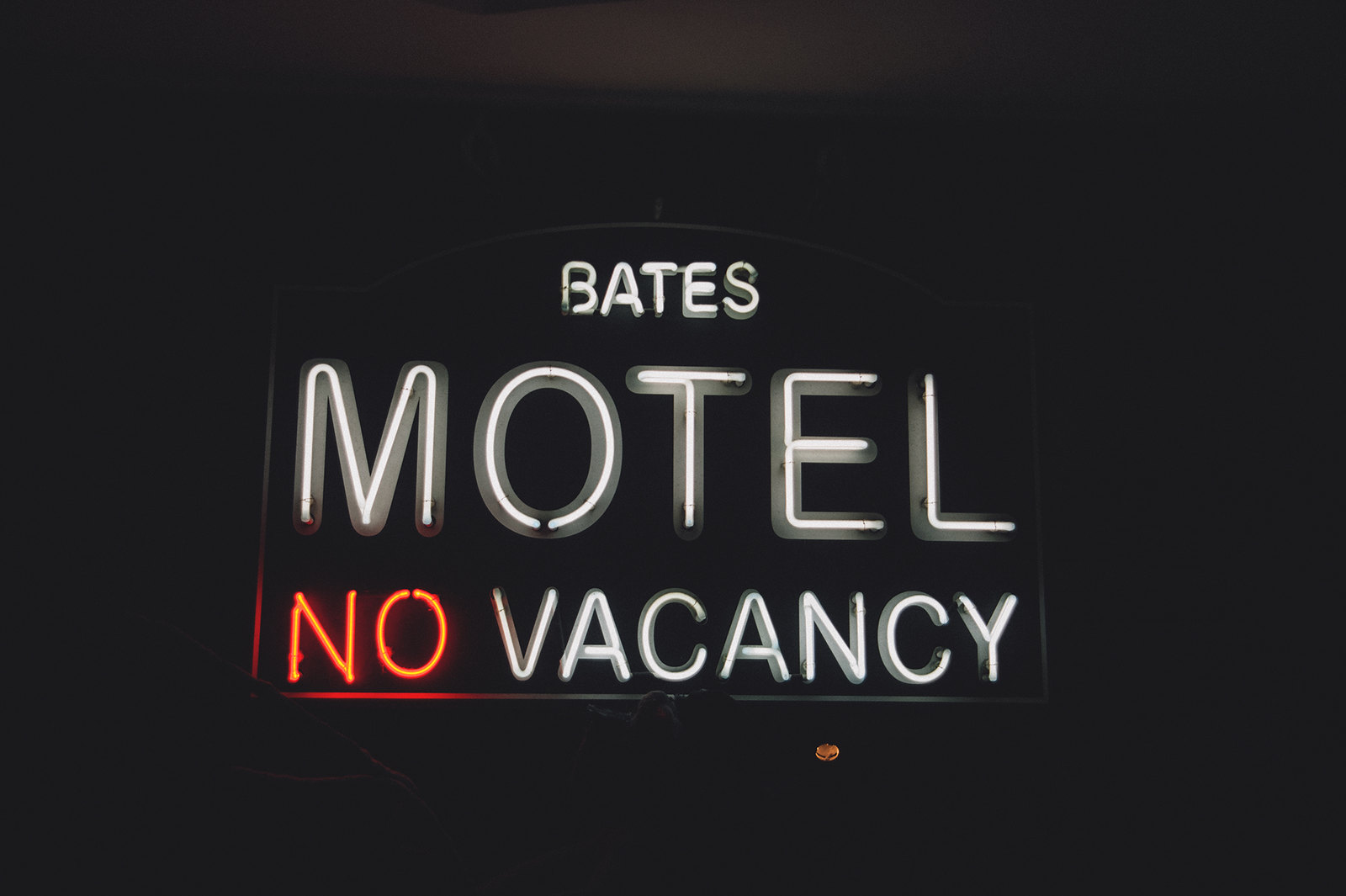In this predominantly black photograph, a neon sign commands attention at the center. The sign, illuminated against the pitch-dark background, reads "BATES" in small all capital letters followed by "MOTEL" in much larger all capital letters. Beneath this, the words "NO VACANCY" are displayed, with "NO" rendered in red neon lights and "VACANCY" in white. The sign takes up approximately 30% of the image, with the dim outlines of possible figures scarcely visible beneath the letters, specifically under the "C" in "VACANCY." The top middle section of the image shows faint whitening, adding a subtle contrast to the otherwise dark scene. Below "VACANCY," a circular object in a golden color is faintly discernible, though hard to clearly identify.